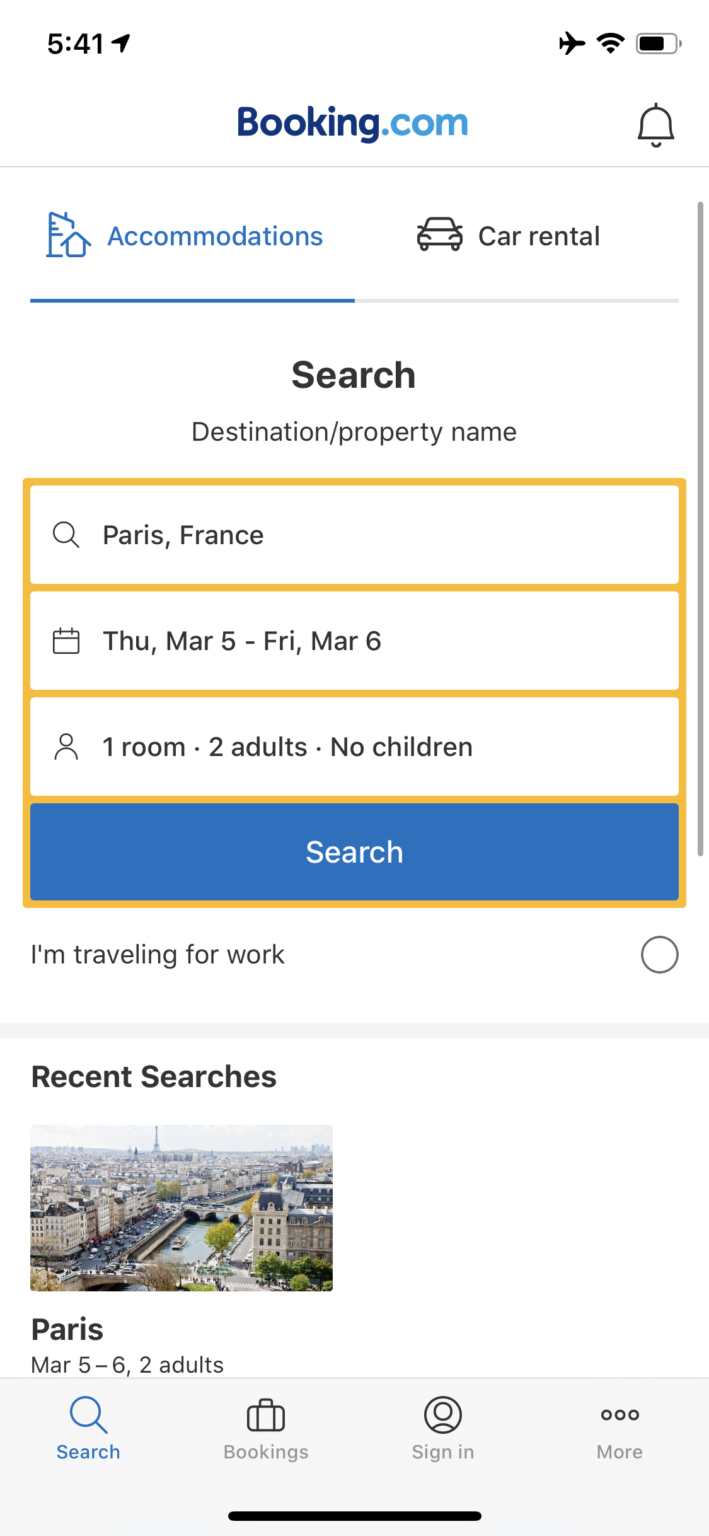A mobile phone screen displaying a section of the Booking.com interface is prominently shown. The top of the screen indicates the time is 5:41. Location services are active, represented by a paper airplane icon pointing to the northeast. Additionally, icons show that the phone is in airplane mode with Wi-Fi on, a good Wi-Fi signal, and an 80% battery charge.

At the top of the interface, "Booking" is written in dark blue text with ".com" in a turquoise blue. A notification bell is present, but there are no current notifications indicated. Below this, a faint gray line segments the interface, leading to two selectable options: "Accommodations" and "Car Rentals." The "Accommodations" option is highlighted in blue with a corresponding icon of a house and hotel, while "Car Rentals" is grayed out with a car icon beside it.

Further down, a search area is displayed. The bold black text reads "Search," below which fields prompt the user for "Destination / property name." Three yellow-bordered boxes follow:

1. The first box, containing a magnifying glass icon, reads "Paris, France."
2. The second box, featuring a calendar icon, specifies the dates "Thursday, March 5th to Friday, March 6th."
3. The third box, with a person icon, indicates "1 room, 2 adults, no children."

The search button itself is blue with white text and surrounded by a yellow border, consistent with the other input boxes. Below the search section, a checkbox labeled "I'm traveling for work" is present but not selected.

A thicker gray line separates this area from the "Recent Searches" section. This section showcases a thumbnail image of Paris, depicting a body of water, the Eiffel Tower, and surrounding buildings. Accompanying text states "Paris March 5th to the 6th, 2 adults."

At the bottom of the screen, a gray navigation bar features four icons:
1. A blue magnifying glass for the focused "Search" section.
2. A gray suitcase labeled "Bookings."
3. A person icon within a circle for "Sign In."
4. Three horizontal ellipses for "More" options, all above a prominent thicker oval underline.